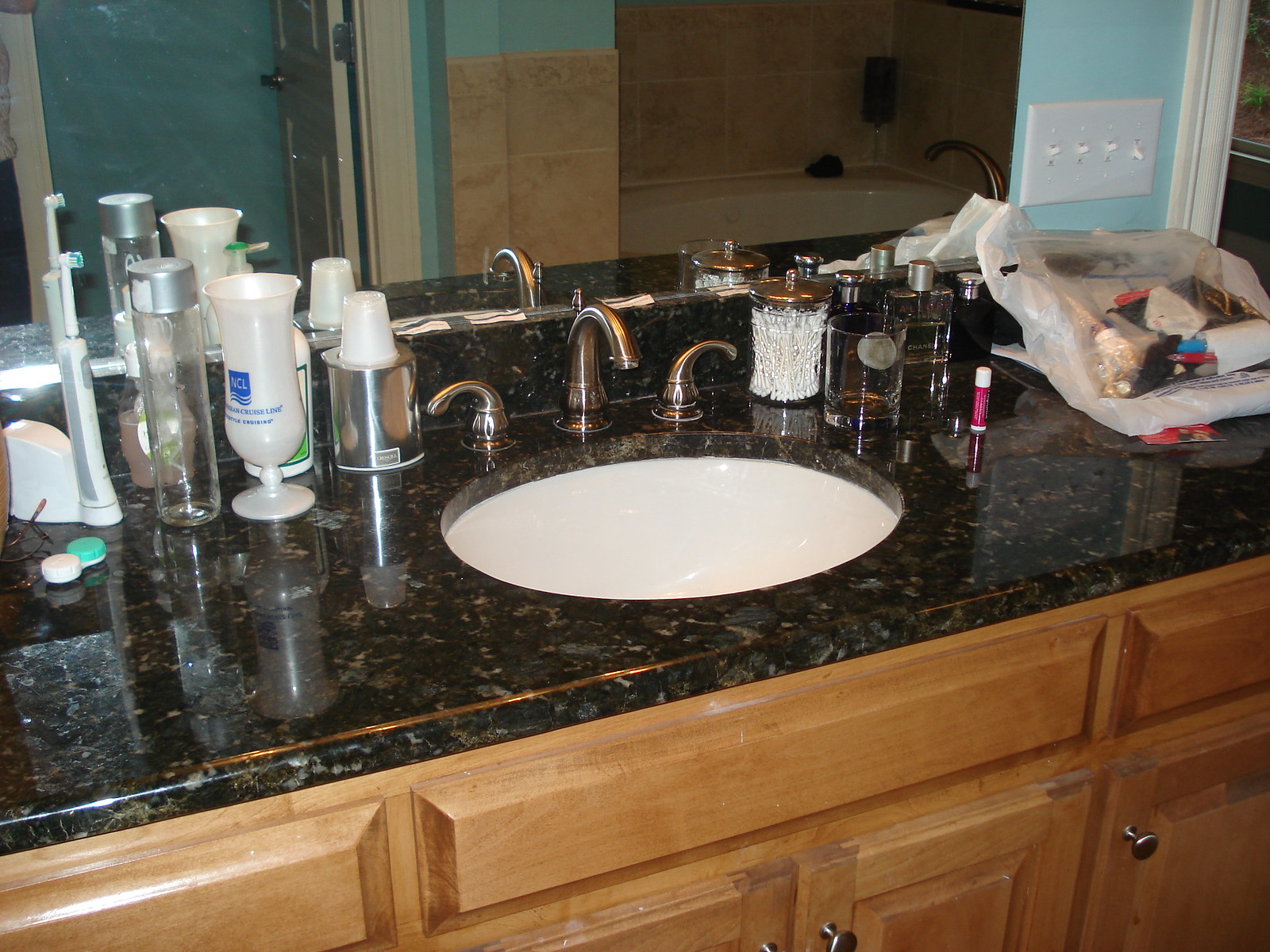This image depicts an elegant bathroom vanity crafted from black and gold marble. The focal point is a round sink, complemented by a faucet that arches gracefully over it, accompanied by hot and cold water handles that curve similarly. The vanity surface is adorned with various personal items, including a chapstick, a glass container filled with cotton swabs, a glass that may contain liquid, a bottle of cologne, a contact lens case, a pair of glasses, and an electric toothbrush. Additional items include a clear bottle, a white glass, and a small silver container holding disposable glasses. On the far right side, a bag lies with several items resting on it. 

Above the vanity, a light switch panel with four switches is mounted on a wall painted in a bluish-green hue. A large mirror stretches across the back of the vanity, reflecting a bathtub surrounded by tan-colored tiles in the background. The mirror also captures the reflection of an open door on the left side, painted in the same bluish-green as the wall behind the light switch panel.